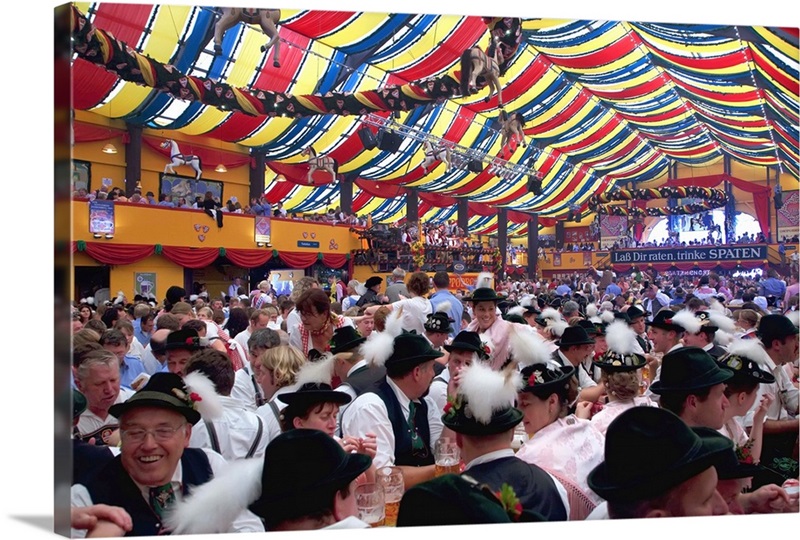The photograph captures a bustling scene inside a brightly colored Oktoberfest tent. The tent is adorned with alternating stripes of red, yellow, and blue, along with thinner black and white translucent stripes to allow sunlight to stream in. At the far end of the tent, there's an archway letting in more sunlight, and a blue banner featuring white German text, which appears to read “Labdirraten Trinken Spaten” or something similar. 

The large crowd is packed shoulder-to-shoulder, giving the impression of a lively, festive atmosphere. Many attendees are dressed in traditional German attire, with men wearing black hats, black vests, and long-sleeved white shirts, while some women also sport black hats. The tables are lined with tall glasses of brown beer, adding to the festive Oktoberfest vibe. The left wall of the tent is an orange-ish hue, adding warmth to the overall scene. This detailed depiction showcases the communal and celebratory essence of the event.